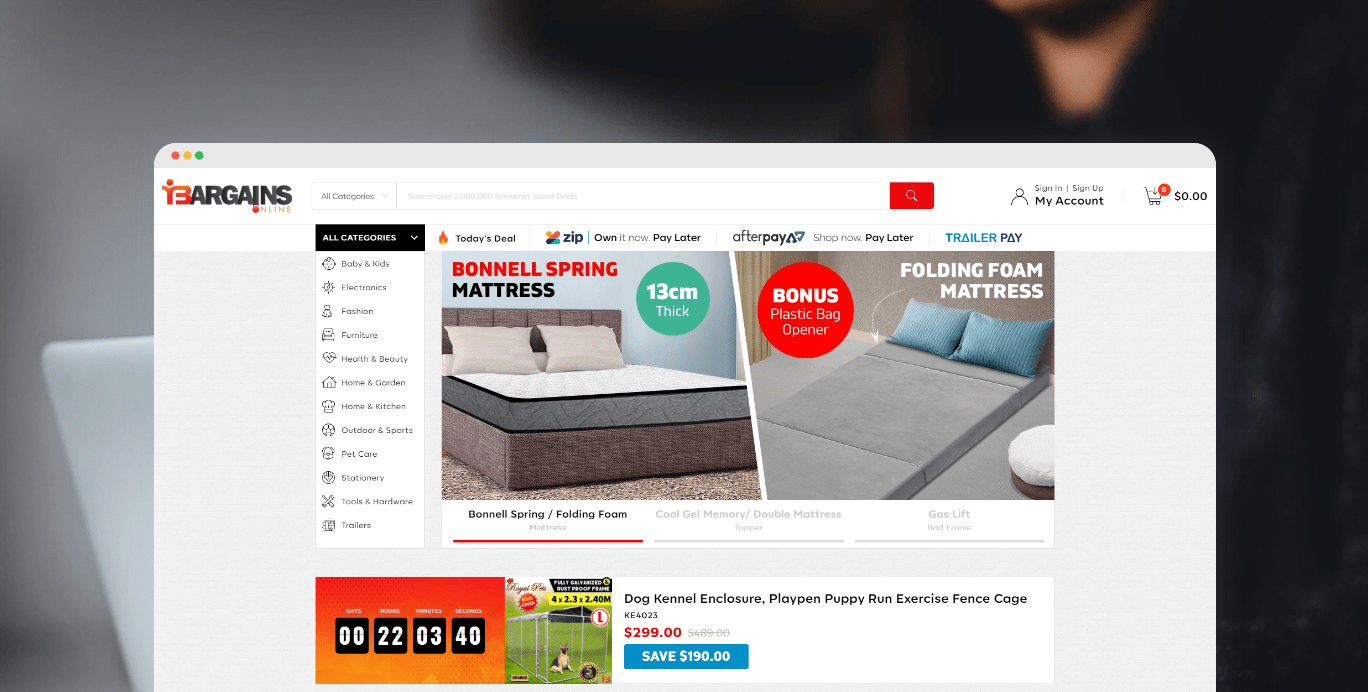The image is a screenshot of an online storefront, characterized by a clean and minimalist design in shades of gray and white. In the background, there's a slightly blurred image of a person in a black outfit standing against a gray backdrop, with a white chair to the left.

At the top left corner of the website, three small dots in red, yellow, and green are displayed. Below these dots, the website's name, "Bargains Online," is prominently featured, accompanied by an "All Categories" dropdown menu and a search bar highlighted by a red block with a white magnifying glass icon. On the top right corner, user options such as "Sign In," "Sign Up," "My Account," and a shopping cart icon showing "$0" are visible.

The main navigation menu lists a variety of categories: All Categories, Baby and Kids, Electronics, Fashion, Furniture, Health and Beauty, Home and Garden, Home and Kitchen, Outdoor and Sports, Pet Care, Stationary, Tools and Hardware, and Trailers. Next to these categories, promotional buttons include "Today's Deal," "Zip: Own It Now, Pay Later," "After Pay: Shop Now, Pay Later," and "Trailer Pay."

Highlighted deals on the page include a "Bonnell Spring Mattress, 13 cm thick," that comes with a "Bonus Plastic Bag Opener Folding Foam Mattress." This special offer is available for another 22 hours, 3 minutes, and 40 seconds. Additionally, a "Dog Kennel Enclosure, Playpen, Puppy Run, Exercise Vent Cage" is priced at $2.99, offering a savings of $190.